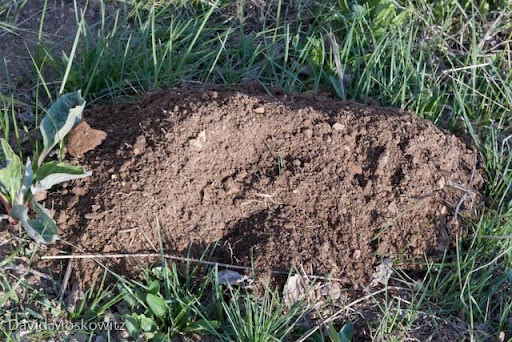The image captures a recent and freshly dug dirt mound positioned centrally on a patch of vibrant, green grass. The dirt is dark brown, with a mixture of small rocks and a slightly patted-down appearance, suggesting recent disturbance possibly by a mole or human activity. The grass surrounding the mound is lush and healthy, with long blades hinting at an outdoor and unmanaged setting. A dandelion weed is visible on the left side, adding to the natural context. The photo, likely taken in the afternoon due to the presence of shadows and sunlight, also features a faint watermark in the bottom left corner, which reads "David Moskowitz."